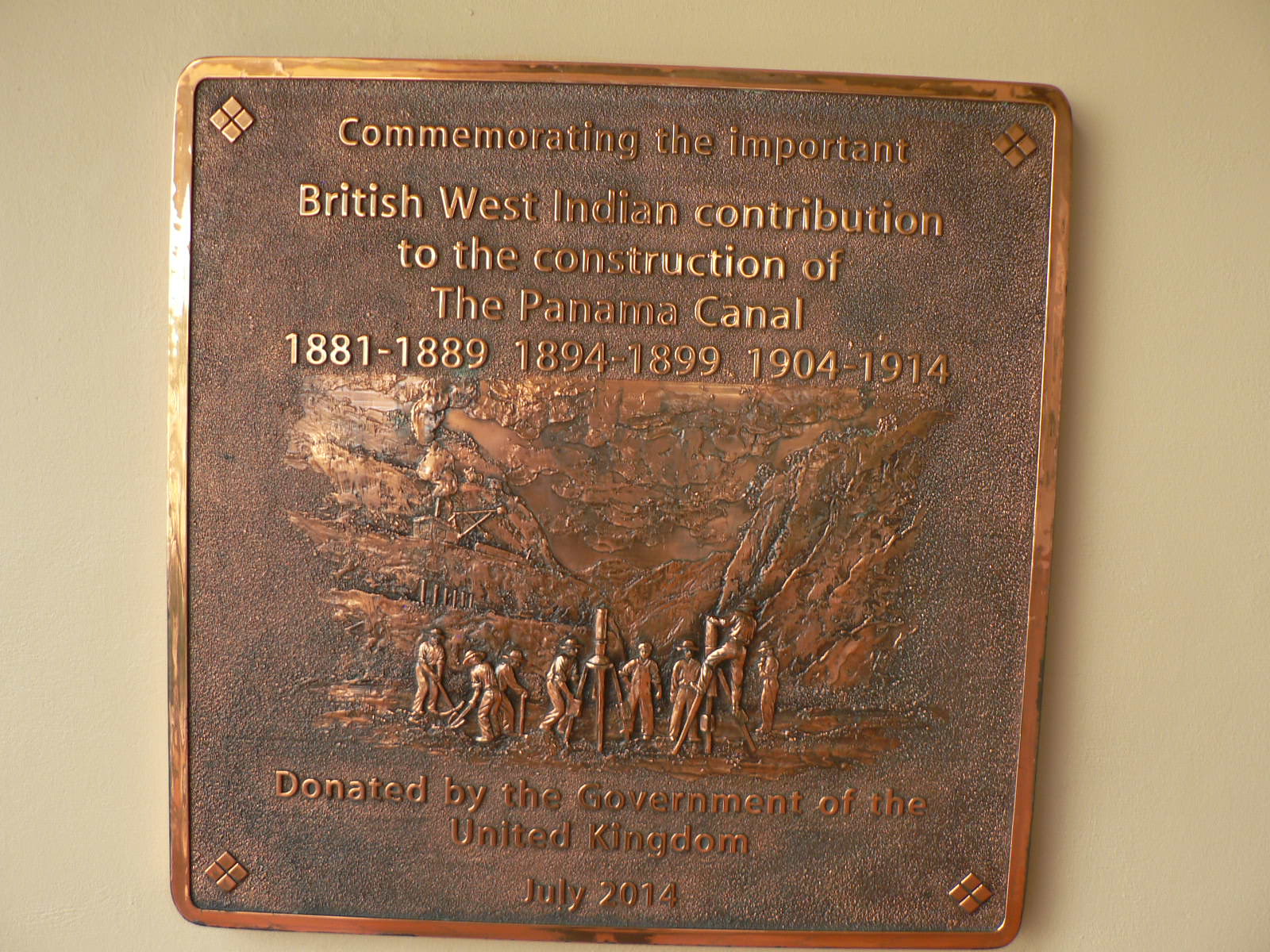This image is a detailed photograph of a bronze-colored plaque mounted on a tan surface. The plaque honors the significant British West Indian contribution to the construction of the Panama Canal across three distinct time periods: 1881 to 1889, 1894 to 1899, and 1904 to 1914. The top of the plaque bears the inscription commemorating this contribution, while the bottom states it was donated by the government of the United Kingdom in July 2014. Centrally featured is an engraved depiction showing several West Indian workers engaged in canal construction, with their surroundings possibly representing the canal or nearby mountains. The image appears slightly worn, suggesting age or exposure. The photograph itself is angled, providing a perspective view that adds depth to the portrayal. It’s uncertain if the setting is indoors or outdoors, or whether it was taken during the day or night. The background is a uniform tan, making the plaque's distinctive bronze and engraved details stand out.